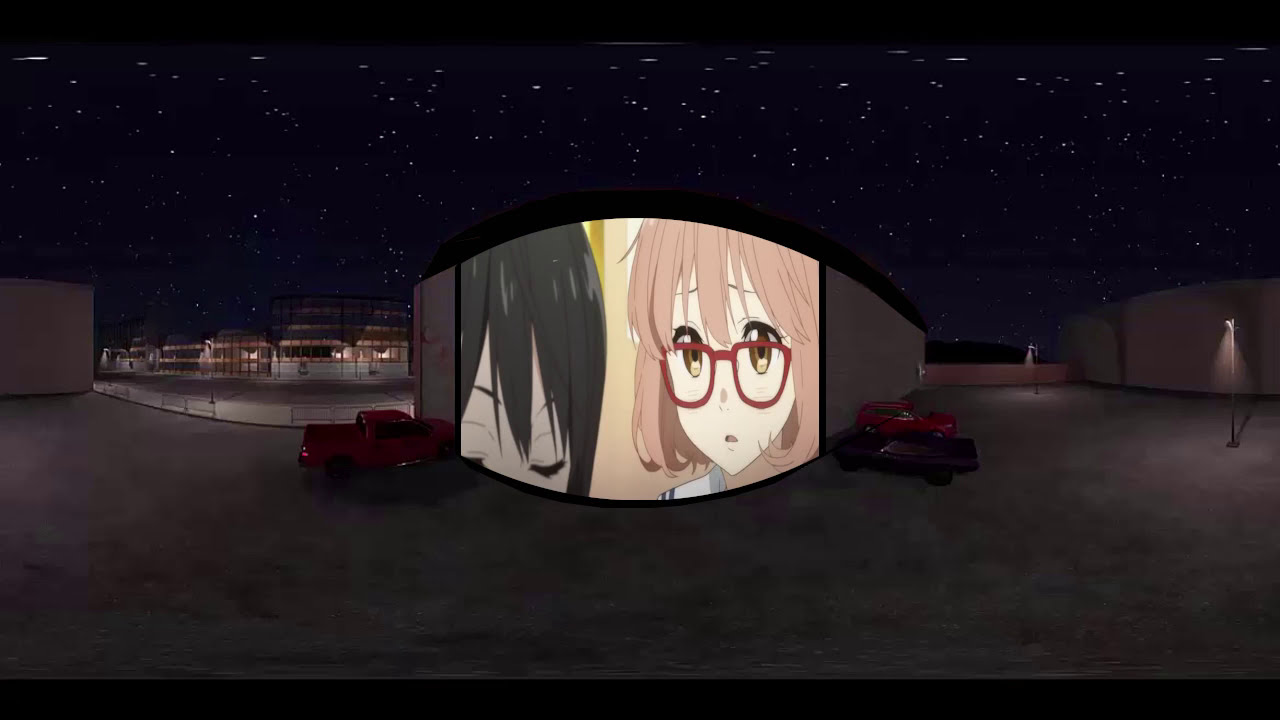The image is a horizontally aligned rectangular nighttime photograph depicting a scene reminiscent of a drive-in theater. The upper and lower parts of the photo are bordered by thick, black spaces framing the central subject: a curved screen that is displaying an anime or cartoon movie. The main character on the screen is a young female with short brown hair, bangs, and red glasses. She has large brown eyes and an expression of surprise, her mouth forming an 'O' shape. Next to her on the screen is another female character, distinguishable only by her black hair and closed eyes.

The background features a solid black sky adorned with tiny white stars, adding to the nighttime ambiance. In front of the screen and stretching across a large cement area, there are several vehicles parked as if at a drive-in. On the left side of the screen, a red pickup truck is parked, while on the right side, an older sports car is accompanied by a red SUV. The backdrop includes a fence, contributing to the outdoor setting, and there are blank screens extending further along the curve of the primary screen. The scene is devoid of text, and the colors in the image primarily include black, gray, red, white, pink, beige, and tan.